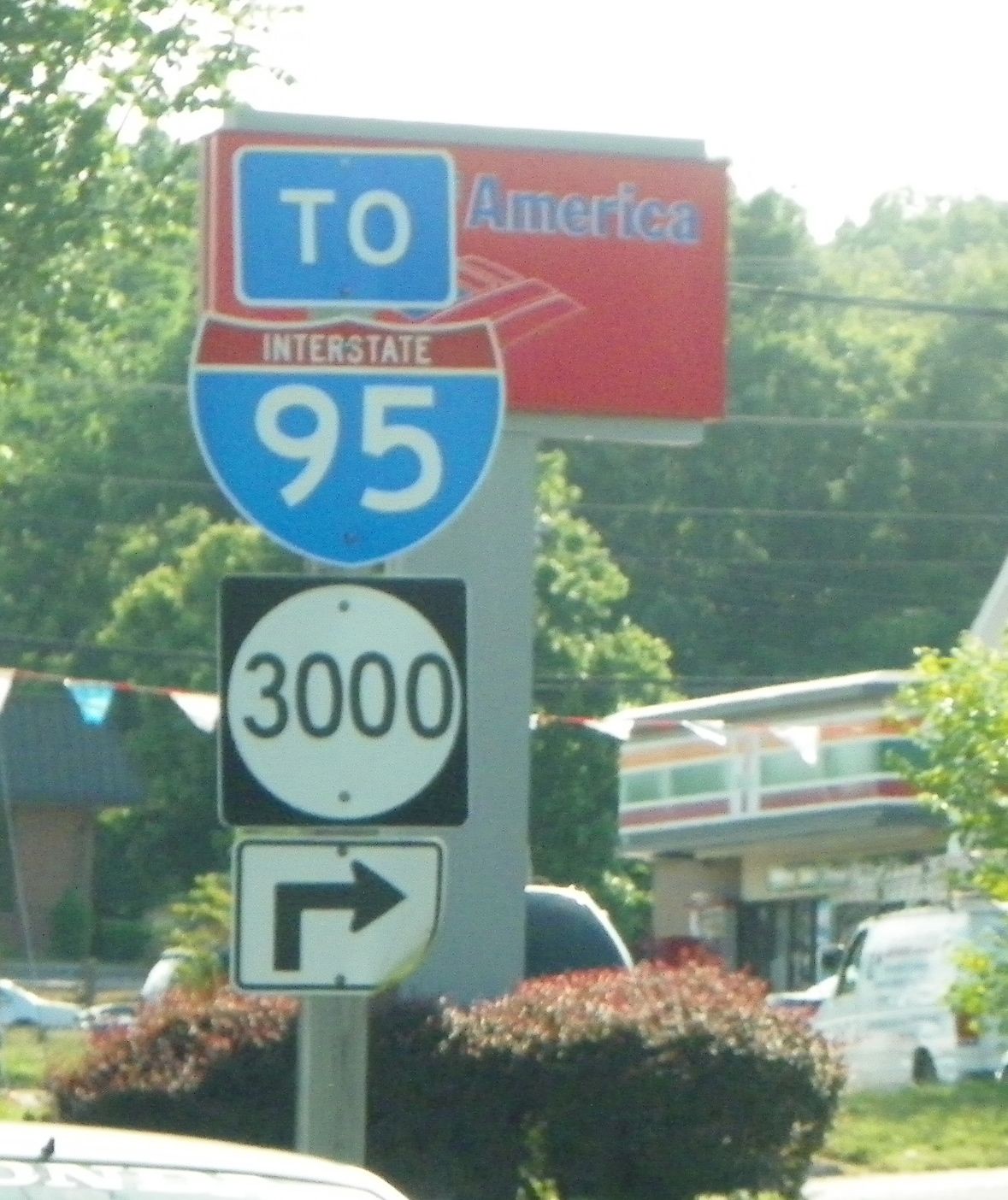The photograph captures a streetscape featuring multiple signs. Prominently, a street sign directs traffic towards Interstate 95. Below it, another sign displays the number "3000," though its significance is unclear. Additionally, a directional sign with a right arrow indicates a turn. In the background, the familiar logo and storefront of a 7-Eleven convenience store are visible. The juxtaposition of the signs and the store provides a sense of urban navigation and commercial presence.